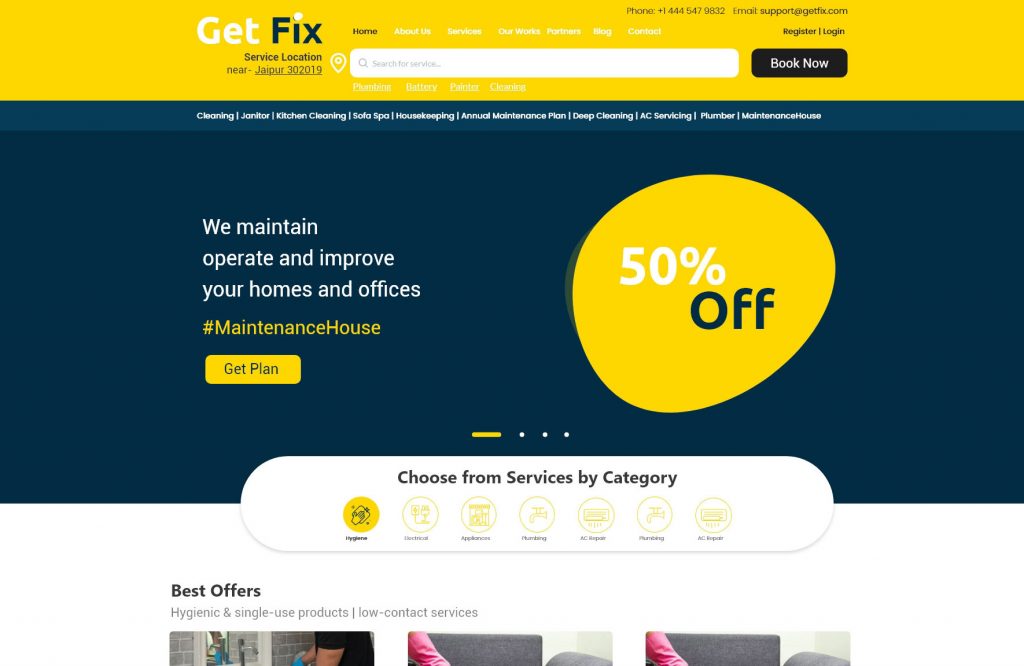This is a detailed copy of a screenshot of a webpage with a vibrant design. At the top, the header boasts a striking yellow background. The brand name, "Get Fixed," is prominently displayed with the text in white and blue hues. Just below "Get Fixed," the service location is specified as "near Jaipur, 302019."

On the right side, there is a navigation menu featuring "Home" in blue, with other menu options such as "About Us," "Service," "Our Work," and three additional items in white. Just below this menu, a search box is visible along with a "Book Now" button. Above this section, options for "Register" and "Log In" are present, and even higher up, the company's phone number and email address are listed.

In the body of the page, a sub-menu offers various selections. The main image features a bold dark blue background with the text "We Maintain, Operate, Improve Your Home and Offices" prominently displayed in white. Accompanying this message, there is a hashtag "#maintenance" and "#house," along with a yellow button labeled "Get Planned."

To the right of this section, an oval-shaped badge announces "50% Off." Below this, another oval includes circular options under a label "Choose Service by Category."

Further down, a header labeled "Best Offers" is followed by three partially visible images. Directly beneath this header, descriptive text reads, "Hygienic and Single-Use Products, Low Contact Service."